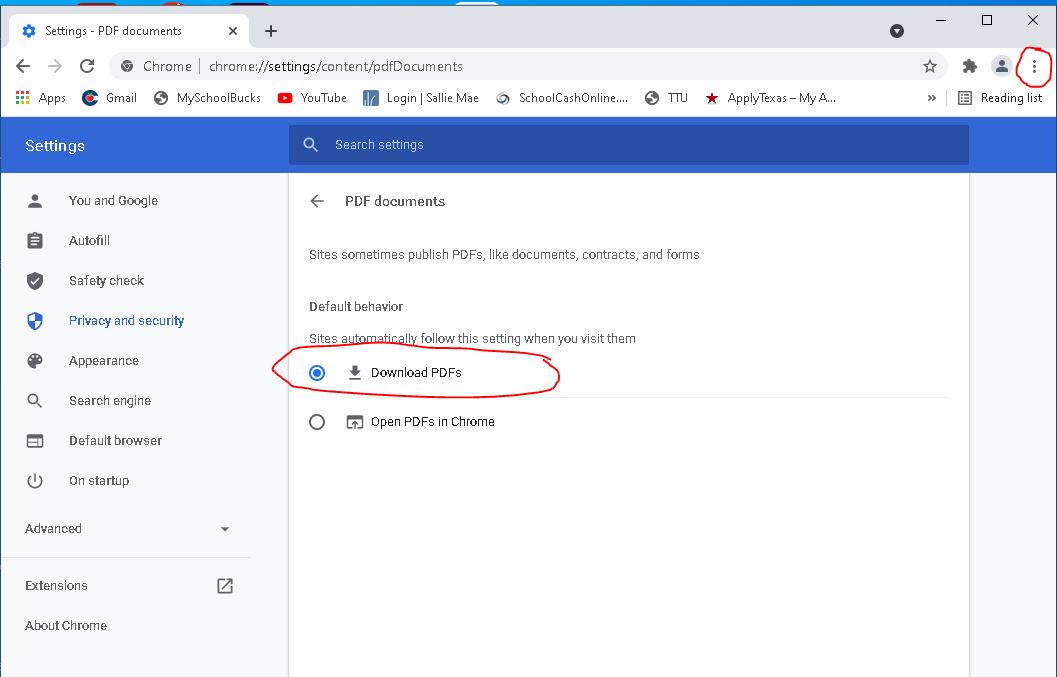**Detailed Caption:**

The screenshot depicts a browser window open to a specific settings page within Google Chrome, indicated by the URL "chrome://settings/content/pdfDocuments" in the address bar. The page focuses on settings related to PDF documents.

The settings page showcases two primary options for handling PDFs:
1. "Download PDFs" is highlighted in blue, signifying that it is enabled. This option is further emphasized with a hand-drawn red circle around it.
2. "Open PDFs in Chrome" remains unchecked and is not circled.

Below the address bar, a bookmarks bar lists several frequently used links including:
- Apps
- Gmail
- MySchoolBucks
- YouTube
- Login
- Sallie Mae
- School Cashout Online
- TTU
- Apply Texas
- Reading List

To the right, three vertical dots, representing a menu, are circled in red. This menu typically provides additional options or settings.

On the left side of the settings page, navigational links appear, including:
- Settings
- You and Google
- Autofill
- Safety Check
- Privacy and Security
- Appearance

The image has annotations, likely added with a photo editor, to highlight and instruct on specific settings. The hand-drawn circles in red serve to draw attention to critical elements: the "Download PDFs" option and the vertical three-dot menu.

This screenshot appears to be part of a tutorial, guiding users on how to configure PDF handling settings in Chrome.